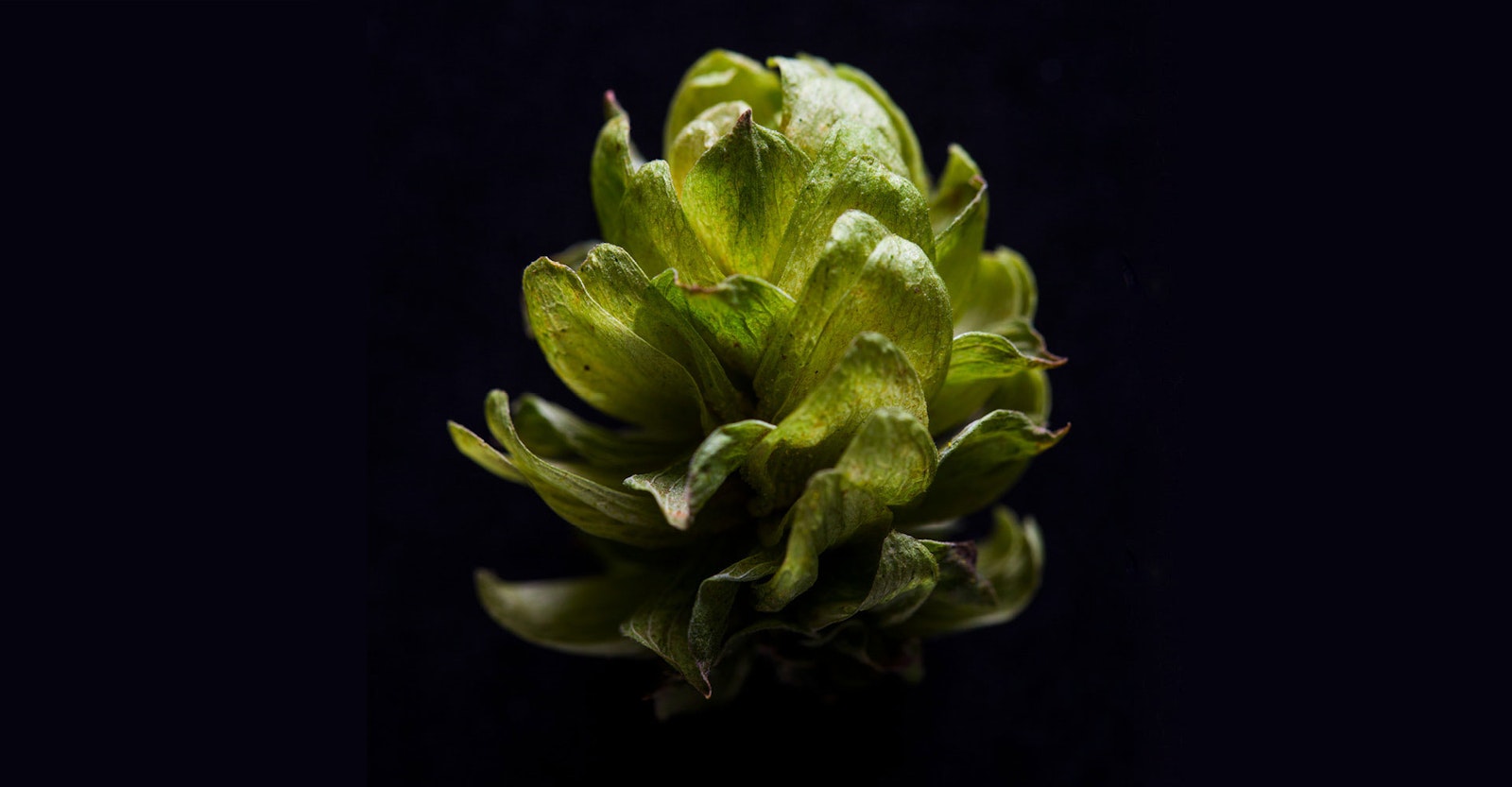The image showcases a plant with a completely black background, illuminated by a distinct light source from the upper right. The light accentuates the medium-toned green leaves, which are arranged in layers reminiscent of both an artichoke and a pine cone. The leaves exhibit a high level of detail, appearing somewhat shiny and veiny under the bright light. The plant's leaves are small and somewhat rounded with a slight point at the tips, some of which display a singed or toasted brown and black edging. The leaves fan out in different directions: leftward on the left side, upward and curling in the middle, and outward to the right, creating a dynamic yet orderly appearance. The entire composition centers on this plant, with the stark black background emphasizing the vibrant, intricate foliage.